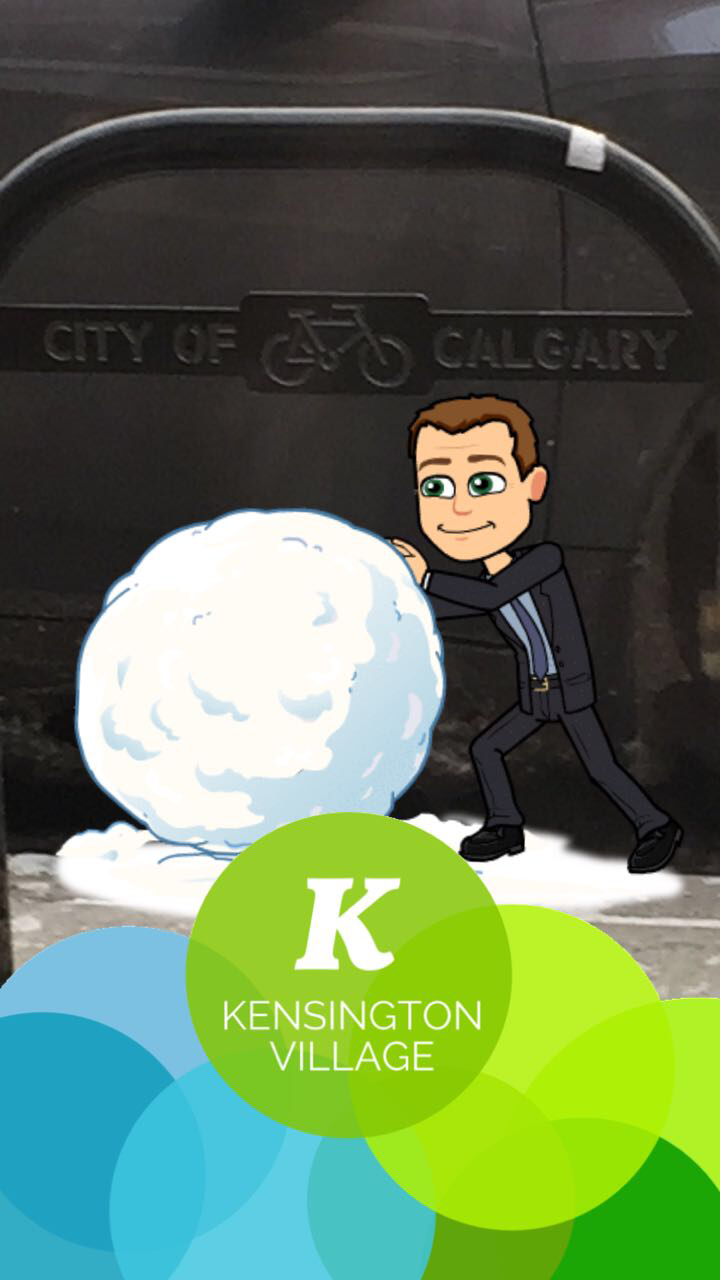In the image, there is a prominent cartoon character depicted with short brown hair and large green eyes. The character has a square face and is dressed in a black suit, a blue undershirt, and a blue tie. He is energetically rolling a giant white snowball. The background features a mix of real-life objects and elements, including a black steel bar and a gray bicycle. Additionally, there's a black bag placed nearby. Beneath these elements, there is a light green circle with a white letter "K" and the text "Kensington Village" below it. The background is also adorned with overlapping circles in various shades, including light green, blue, dark blue, and dark green, creating a cohesive patterned design. The cartoon character is centered amidst these diverse elements.